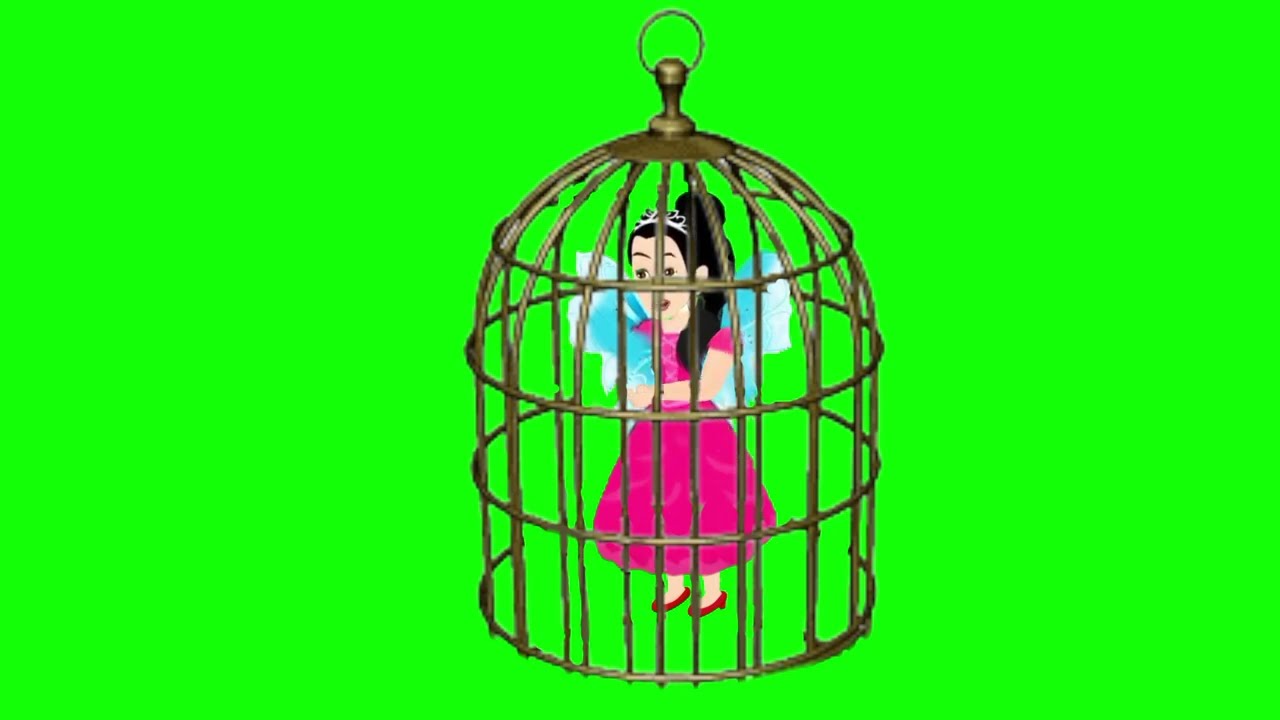The image showcases a vivid, neon lime green rectangular background, with a gold metallic birdcage prominently placed in the center. The cage, designed with a ring at the top, stands freely with no bottom, appearing open at the back. Inside the domed, bird-like cage is a cartoon depiction of a woman with long black hair flowing down to her left shoulder. She is adorned with a silver tiara and a short-sleeved, flowing pink ball gown. Her feet are encased in red shoes reminiscent of Dorothy's slippers from the Wizard of Oz, and she has light blue wings outlined in white extending from her back. She stands with her arms folded and hands clasped, her expression slightly open-mouthed as she seems to gaze outward. This vibrant and whimsical scene evokes a sense of delicate captivity within a fantastical, fairy-tale setting.